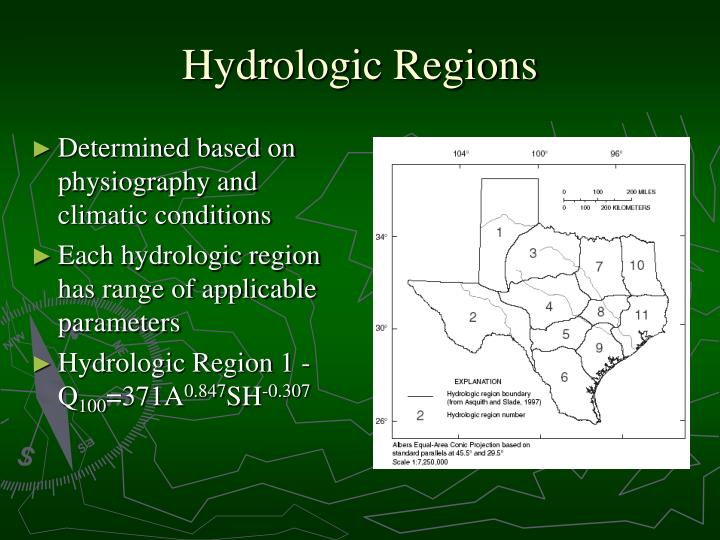The image is titled "Hydrologic Regions" and features a map drawing in black on a simple white background, which is placed on a green background filled with text information. To the left, there are three bullet points written in white font and marked by lime green triangles pointing inward. These bullet points state: "Determined based on physiography and climatic conditions," "Each hydrologic region has a range of applicable parameters," and "Hydrologic Region 1 - Q₁₀₀ = 371A⁰.⁸⁴⁷ SH⁻⁰.³⁰⁷." Behind the map on the green backdrop, there are jagged, scraggly shapes reminiscent of a map, including figures that look like the state of Texas. The coordinates along the map's left edge read 34°, 30°, and 28°, while the top edge reads 104°, 100°, and 96°.